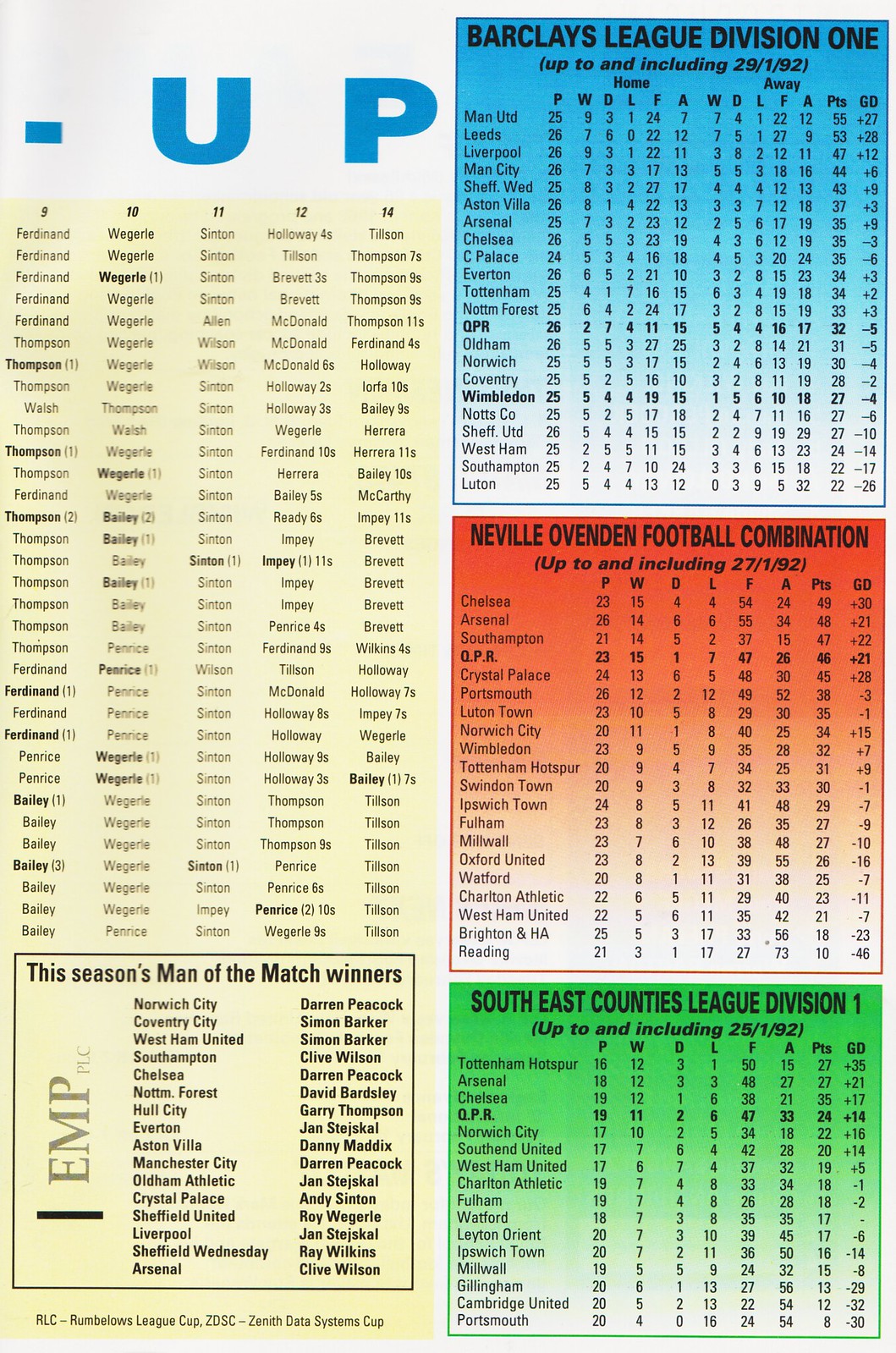The image is a detailed sport information sheet for English football. It is divided into two halves. The right half is further segmented into three sections, each displaying the standings and statistics for different leagues and colored distinctly for clarity. The top section, colored blue, shows the Barclays League Division 1 standings up to and including January 29, 1992, listing all the teams with their home and away scores. The middle section, in red, features the Neville-Ovenden Football Combination standings up to January 27, 1992, similarly displaying the team names and their respective stats. The bottom section, green, details the Southeast Counties League Division 1 standings up to January 25, 1992, also listing various teams and their stats. Additionally, there's a black box that highlights this season's 'Man of the Match' winners, listing out the players' names. The left side of the sheet predominantly includes text in blue capital letters, some names in black type on a white background, and a vertically-oriented text saying "EMP".